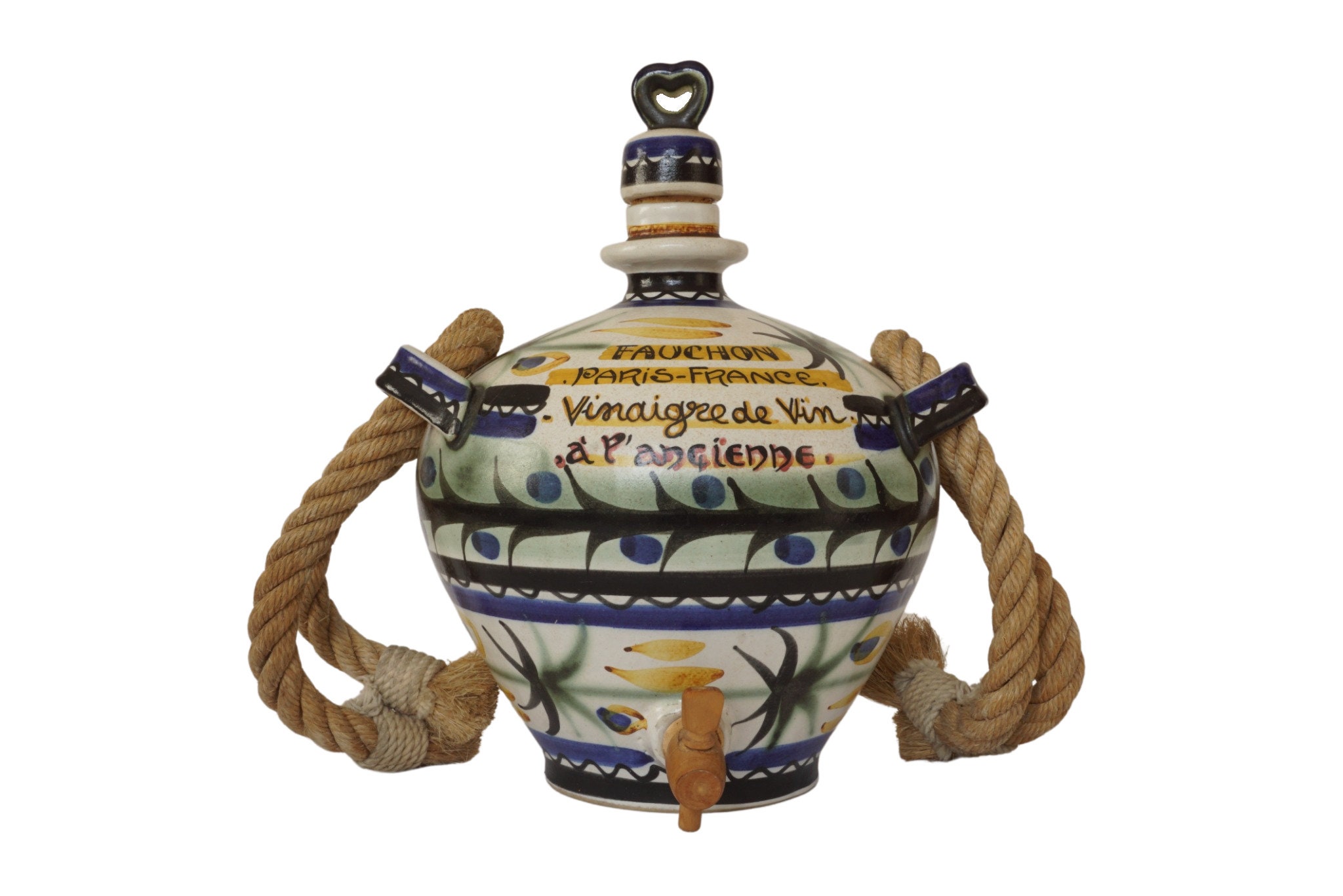The photograph depicts a decorative ceramic water jug with a unique design and vibrant detailing. The jug features a water spout at the bottom, which is equipped with a small faucet-like tap for dispensing liquids. It is adorned with two sturdy, twisted rope handles on either side, secured with smaller ropes to prevent fraying. The jug is topped with a cork stopper, embellished with a black heart. The exterior is predominantly white and beautifully painted with horizontal blue stripes, interspersed with dots and an elegant lace-like pattern. Additionally, there are yellow leaves accentuating the writing and areas above the spout, along with two star motifs on either side of the spout. The jug also features text in French, including "Fauchon, Paris, France," suggesting it might have been used for storing vinegar or another type of liquid. This container's elaborate decoration and functional design make it a striking and practical piece.